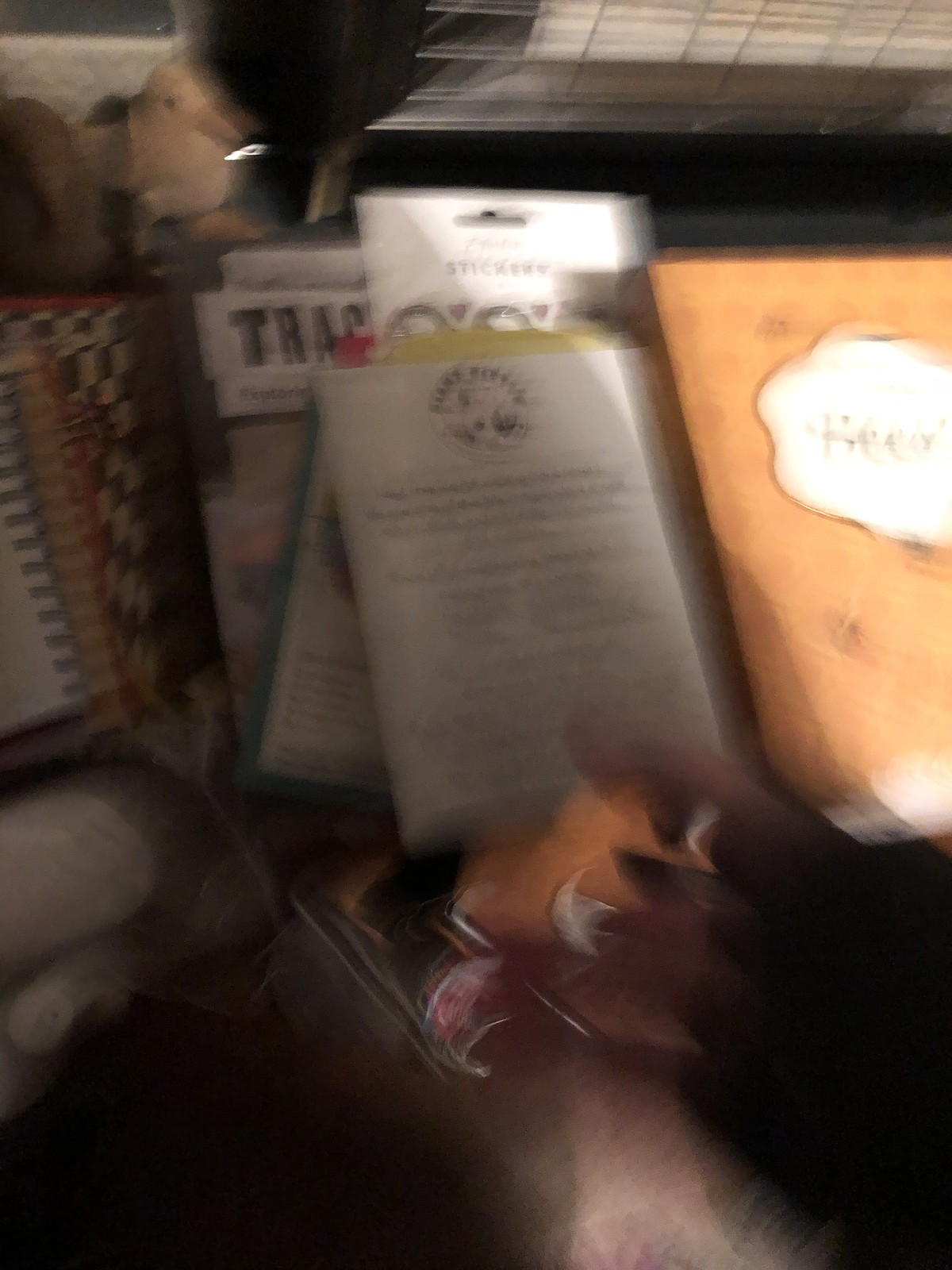In this highly out-of-focus photograph, we're looking downward at a cluttered scene with various items, primarily books and packaging. The background in the bottom left and right corners is black, creating a stark contrast to the faintly illuminated items in the center. There are a few spiral-bound notebooks on the left side; one with a blue spiral and another with a red spiral. There's also a checkered pattern visible underneath them. Beyond the notebooks, on the far left, there's a stuffed animal, possibly a duck given its yellow color and orange beak. 

The center of the image is slightly clearer, showcasing a mix of flat-packaged products. The main item here appears to have a white front with some unreadable text and a circular clip for hanging, hinting it might be instructions or sticker sheets. Below it, another package with a dark green outer edge is visible, layered over others. An orange book, potentially bearing the word "Recipes," is positioned on the far right, made more indistinguishable by light casting from the right. 

In the upper corners, you can spot some wire baskets or cables adding to the chaotic scene. Overall, despite the blurriness, you can discern a mix of colorful spirals, various packaging, and an assortment of books, all amid scattered light and shadow, contributing to the photograph's dynamic yet disorganized composition.